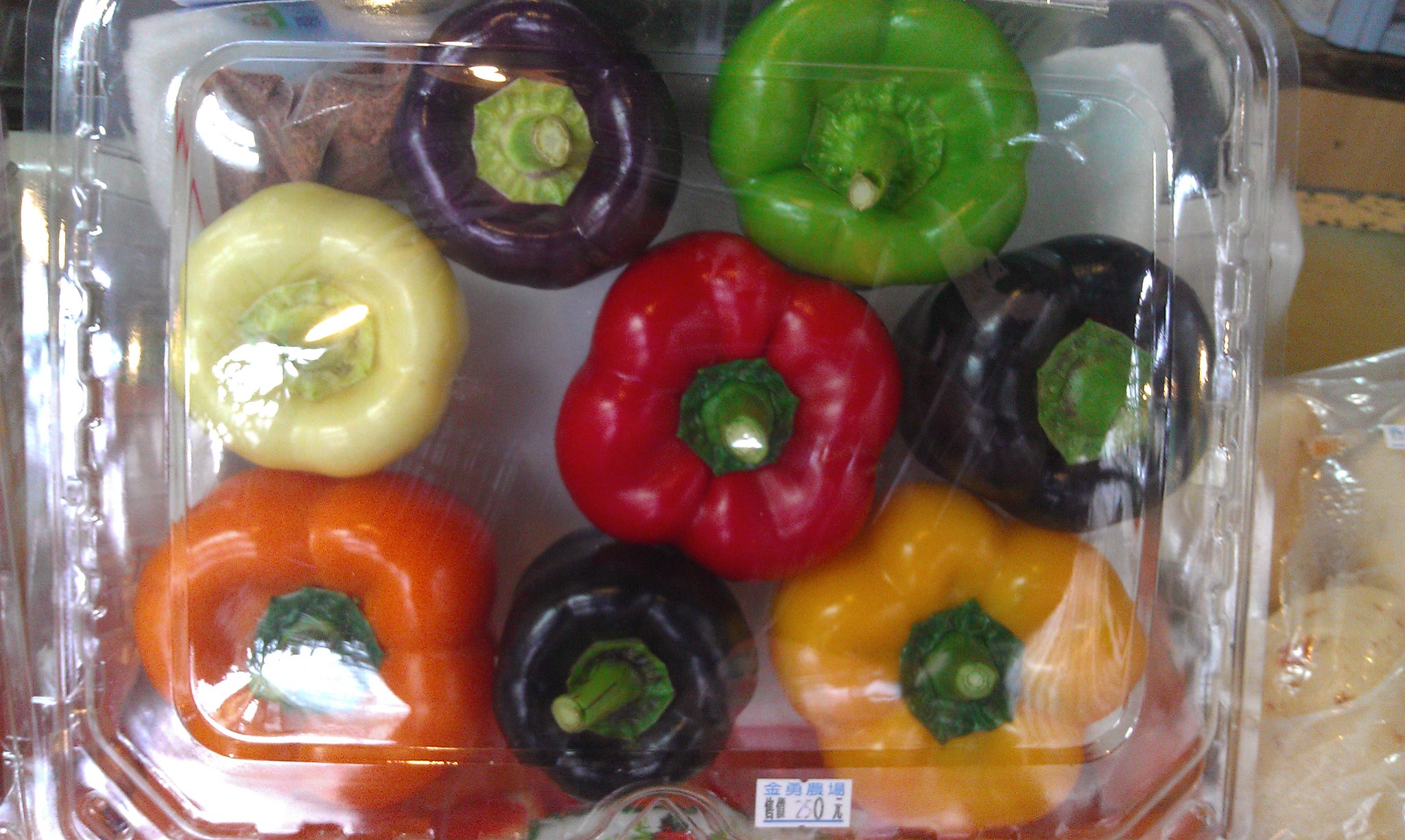This image, photographed from above, features a see-through plastic clamshell package filled with eight bell peppers of various unconventional colors. The package occupies the majority of the frame, set on an indistinct flat surface with noticeable reflections from overhead lighting. The bell peppers are arranged in three rows: the bottom row contains an orange pepper, a dark purple pepper (mistaken by some as black), and a yellow pepper; the middle row includes a creamy off-white pepper on the left, a red pepper in the center, and another dark purple pepper on the right; the top row has a purple pepper on the left and a bright green pepper on the right. Each pepper retains a green stem cut about half an inch above, indicating their freshness. A price tag with blue lettering, difficult to fully decipher but possibly reading '250', is placed prominently in the center of the package. Additionally, a plastic bag with an unidentified white object appears partially in the frame at the lower right corner.